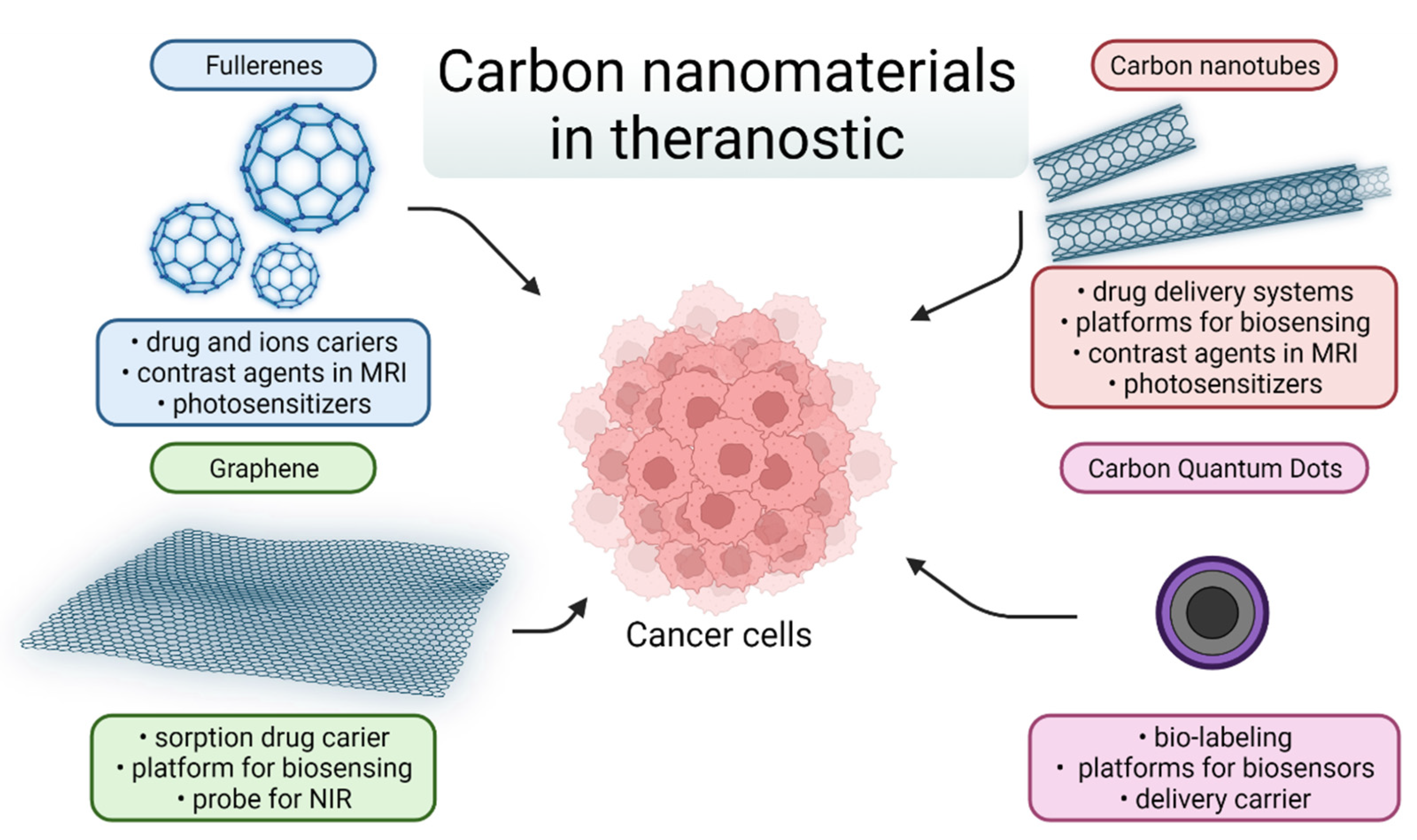**Title: Carbon Nanomaterials in Theranostics**

The infographic provides an in-depth look into how various carbon nanomaterials are utilized in the field of theranostics, with a special focus on their application in cancer treatment. 

At the center of the graphic is a detailed depiction of a reddish-pink cancer cell. The cell is composed of multiple small circles that transition from a light pink outer layer to a darker red inner core, highlighting its complex structure.

To the left of the cancer cell, there is a section dedicated to Fullerenes, represented by a collection of blue spheres. Key points include:
- **Drug and Ion Carriers**: Demonstrating Fullerenes' efficacy in transporting therapeutic agents.
- **Contrast Agents**: Highlighting their role in enhancing imaging techniques.
- **MRI Photosynthesizers**: Denoting their potential use in improving MRI technology.

Beneath this, the section delves into **Graphene**, another significant nanomaterial in theranostics.

On the right side of the graphic, focus shifts to Carbon Nanotubes, depicted visually as intricate, tubular structures. The infographic specifies their applications including:
- **Drug Delivery Systems**: Detailing their capability to effectively convey medication to targeted sites.
- **Platforms for Biosensing**: Showcasing their use in the detection of biological substances.
- **Contrast Agents and MRI**: Reiterating their role in enhancing imaging.
- **Photosynthesizers**: Indicating their utility in photodynamic therapy.

Furthermore, the graphic also addresses **Carbon Quantum Dots**, adding to the comprehensive overview of carbon-based nanomaterials.

Overall, the infographic effectively illustrates the multifaceted roles of carbon nanomaterials in advancing theranostic technologies, particularly in cancer therapy and diagnostics.